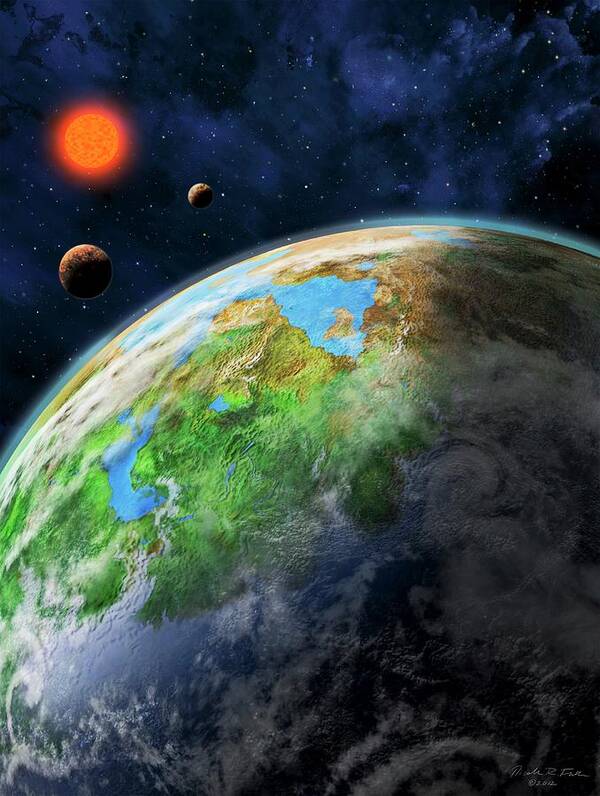The image is an illustration of Earth with other celestial bodies in a galaxy backdrop. The star-filled sky transitions from black to dark blue and purple, creating a vivid and colorful background. An orange and glowing object, likely representing the Sun, illuminates the top left portion of the image, casting light and shading on the other spherical objects. These objects include a reddish-brown and gray orb, possibly depicting another planet or a moon, and a smaller, more distant planet which might resemble Pluto. The Earth is the focal point, shown with a detailed and brightly colored segment of its arc. The illustration highlights green lands, blue waterways, brown deserts, and darker blue oceans, along with white cloud formations. The contrast between the lit areas and darker shaded sections enhances the depth and dimension of the celestial scene. Finally, the painting bears an artist's signature in the bottom right corner, albeit illegible, adding a personal touch to this textbook-like illustration.